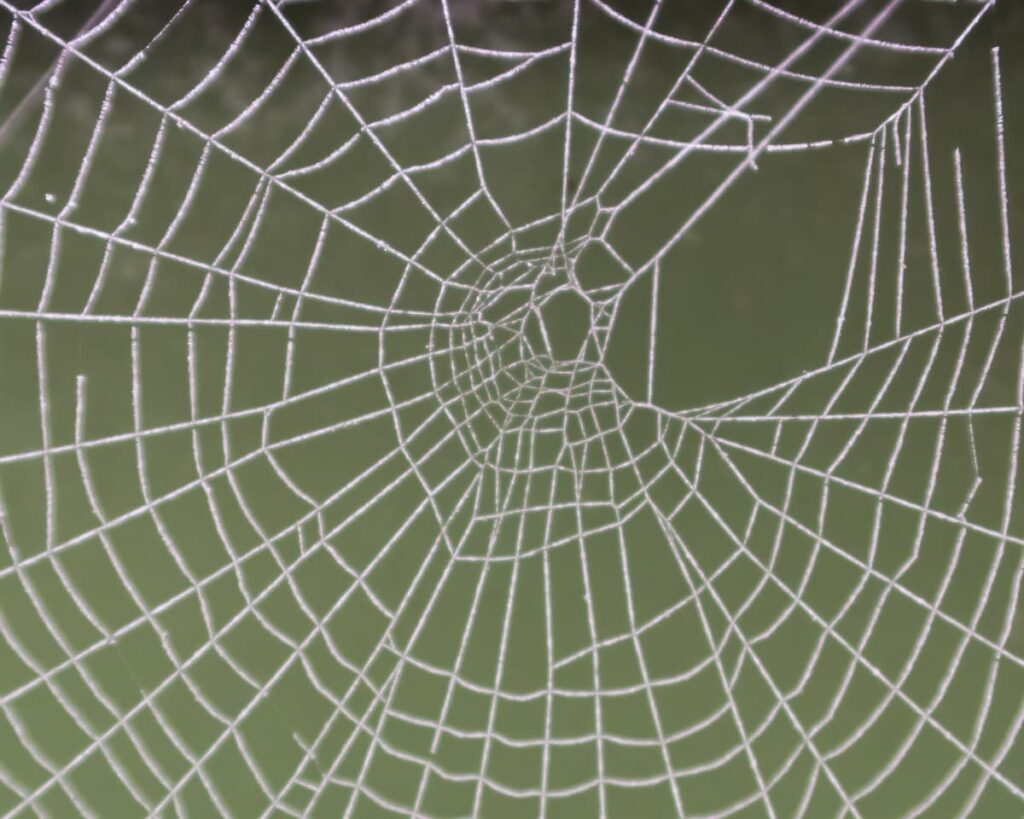This photograph showcases an intricate, funnel-shaped spider web set against a blurred olive green background that transitions to brown near the top. The web is predominantly white, possibly enhanced by morning dew or dust, giving it a striking clarity and a soft, white to beige hue. The pattern of the web is composed of a series of decreasingly smaller rectangles and squares as it funnels inward, designed to trap insects effectively. However, the web shows signs of wear; the right side has a noticeable gap where several cross members are broken, and the left side also has areas with broken silk strands, suggesting interruptions in the web’s construction. The backdrop highlights the delicate beauty and complexity of the spider web, despite its imperfections.